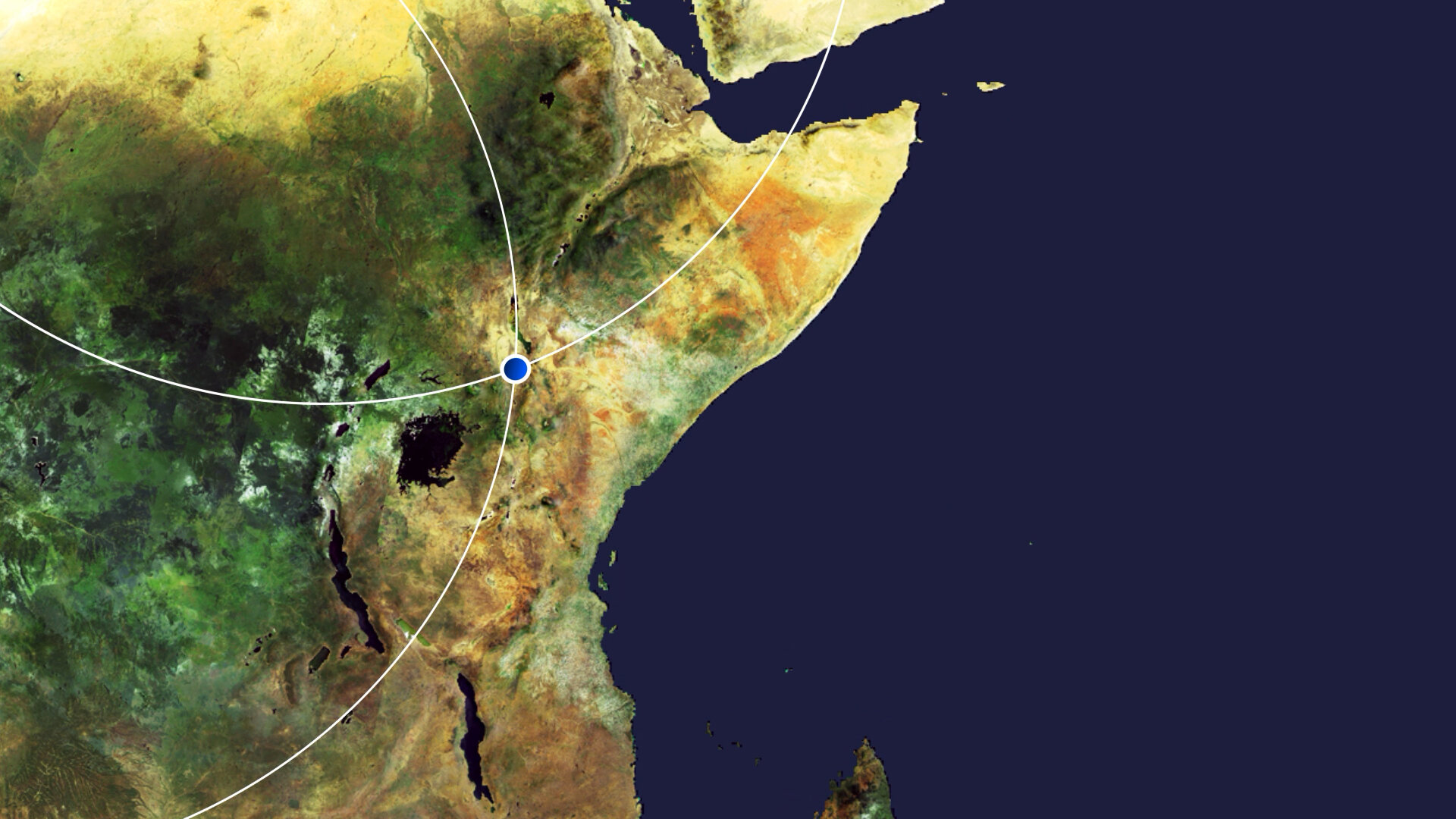This aerial image depicts a detailed map of a region, most likely a part of northeast Africa, with an emphasis on the Horn of Africa bordering the Indian Ocean. The right side of the image is dominated by a deep navy blue color representing the ocean, contrasting sharply with the landmass on the left side. The land features a mosaic of colors, including green areas indicating vegetation, yellow and brown patches signifying desert regions, and hints of orange. Through this land formation, there is a distinct royal blue dot, from which a white line curves up and down, converging at that point, perhaps indicating a point of interest or a specific geographic feature. The jagged and large contours of the landmass, along with the graphic representation, suggest a complex terrain with varying topography and vegetation, captured from a high altitude, providing a comprehensive overview of the region's diverse landscape.